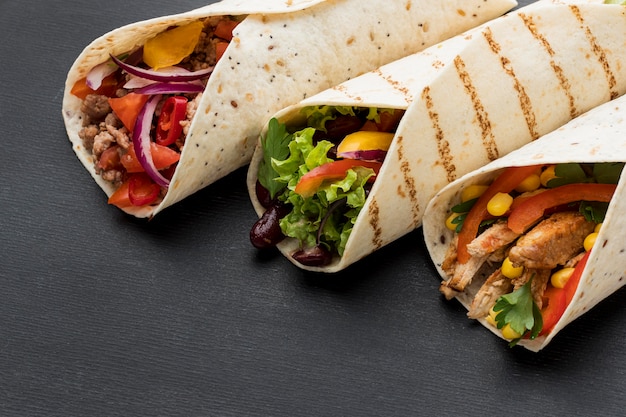The image features three meticulously arranged wraps on a dark, slate-colored, textured surface. Positioned diagonally from the top left to the bottom right, each wrap showcases a variety of colorful, fresh ingredients visible from their open ends. The top wrap, lightly speckled with black pepper or herbs, contains vibrant red onions, chilies, juicy tomatoes, and savory ground meat. The middle wrap, distinct with evenly spaced grill marks, is filled with kidney beans, crisp lettuce, succulent tomatoes, and bright yellow bell peppers. The bottom wrap, similar to the top in appearance, reveals strips of tender chicken, red bell peppers, sweet corn, and fresh coriander. All three wraps are artfully presented under an overhead light, enhancing their appeal on the dark surface below.